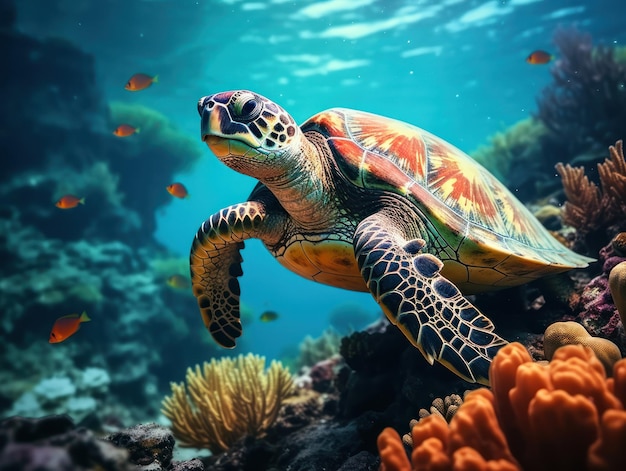This digital art vividly captures an underwater scene featuring a prominently positioned sea turtle. The turtle, highlighted with a detailed orange, yellow, and green shell resembling a tie-dye pattern, displays a sandy tan underbelly and intricately scaled fins that are more navy blue with white lines. The artwork is situated near a vibrant coral reef bed with coral ranging in colors from yellows to oranges, purples, and greens. Surrounding the turtle are various fish, including clownfish and orange fish, enhancing the lively underwater atmosphere. Rock formations and additional underwater flora create depth in the background. Sunlight filters through the cerulean water, casting an ethereal glow over the entire scene, which emphasizes both the natural beauty and the digital craftsmanship of the illustration. The turtle, with a serious expression and defined scales, exudes a tangible realism and charm.